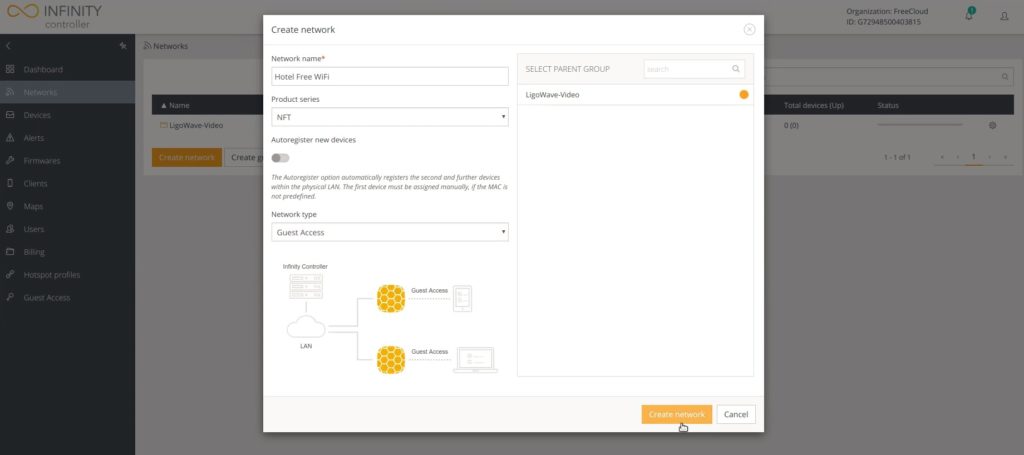In the screenshot, there is a large white pop-up window prominently centered, with the background grayed out. You can still make out some text and graphics on the grayed-out background, including a vertical menu. The menu items are: Dashboard, Networks (which is highlighted), Devices, Alerts, Firmwares, Clients, Maps, Users, Billing, Hotspot Profiles, and Guest Access. Above this menu, there is a yellow infinity symbol next to the text "Infinity Controller."

The pop-up window is titled "Create Network." It contains several fields and options:

- **Network Name:** Entered as "Hotel Free Wi-Fi."
- **Select Parent Group:** With a search bar next to it and the text "LIGOWAVE-VIDEO."
- Next to "LIGOWAVE-VIDEO," there is an orange circle.
- **Product Series:** Listed as "NFT."
- **Auto-Register New Devices:** An option with a slider button that is currently turned off. A description below details that the Auto-Register option will automatically register additional devices within the physical LAN after the first device is assigned manually, provided the MAC is not predefined.

Further down, there is a **Network Type** option set to "Guest Access." Accompanying this option is a diagram showing a flow from "Infinity Controller" to a cloud labeled "LAN," dividing into "Guest Access" at the top and an image of a smartphone connecting to "Guest Access" at the bottom, along with a laptop computer illustration.

At the bottom right corner of the pop-up window, there is an orange rectangle button labeled "Create Network," with a hand pointer icon aiming below it. Adjacent to this button, there is a "Cancel" option.

This comprehensive setup is indicative of a user configuring a hotel’s guest Wi-Fi network through the "Infinity Controller" interface.